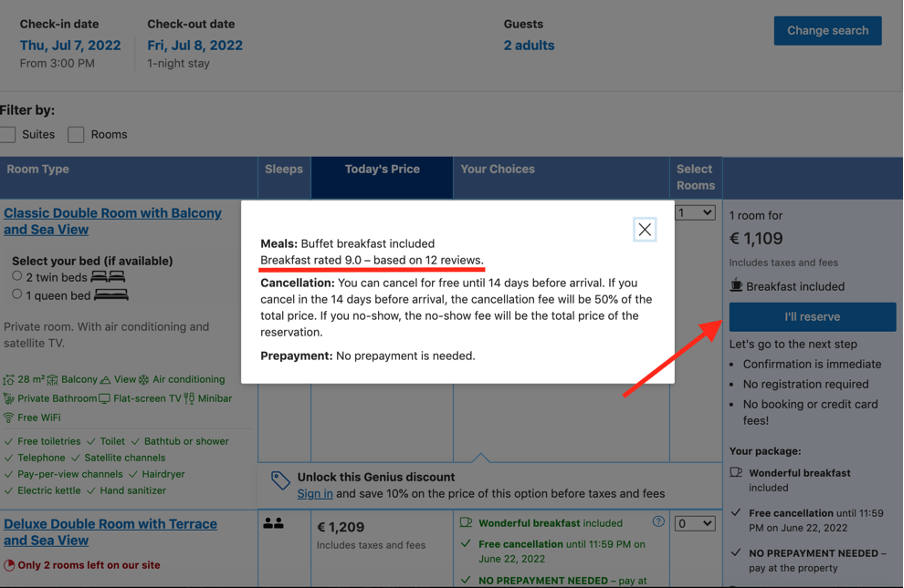On a European hotel or travel website, a user browses accommodation options for a one-night stay from Thursday, July 7th, 2022, to Friday, July 8th, 2022. The user is looking to book for two adults, and the rates are displayed in Euros.

They examine the details of a "Classic Double Room with Balcony and Sea View," where they can choose between two twin beds or one double bed, though no selection has been made yet. The room is described as private, equipped with air conditioning and satellite TV. Highlighted in green are the included amenities: a balcony view, air conditioning, a private bathroom, flat-screen TV, mini bar, free Wi-Fi, free toiletries, toilet, bathtub or shower, telephone, satellite channels, pay-per-view channels, hair dryer, electric kettle, and hand sanitizer.

The user also notices a "Deluxe Double Room with Terrace and Sea View," with only two rooms remaining. However, they opt for the classic double room, priced at 1,100 Euros per night, inclusive of taxes and fees. Breakfast is included with this room type. A blue "Reserve" button allows for quick booking, and an additional button provides details about the included breakfast.